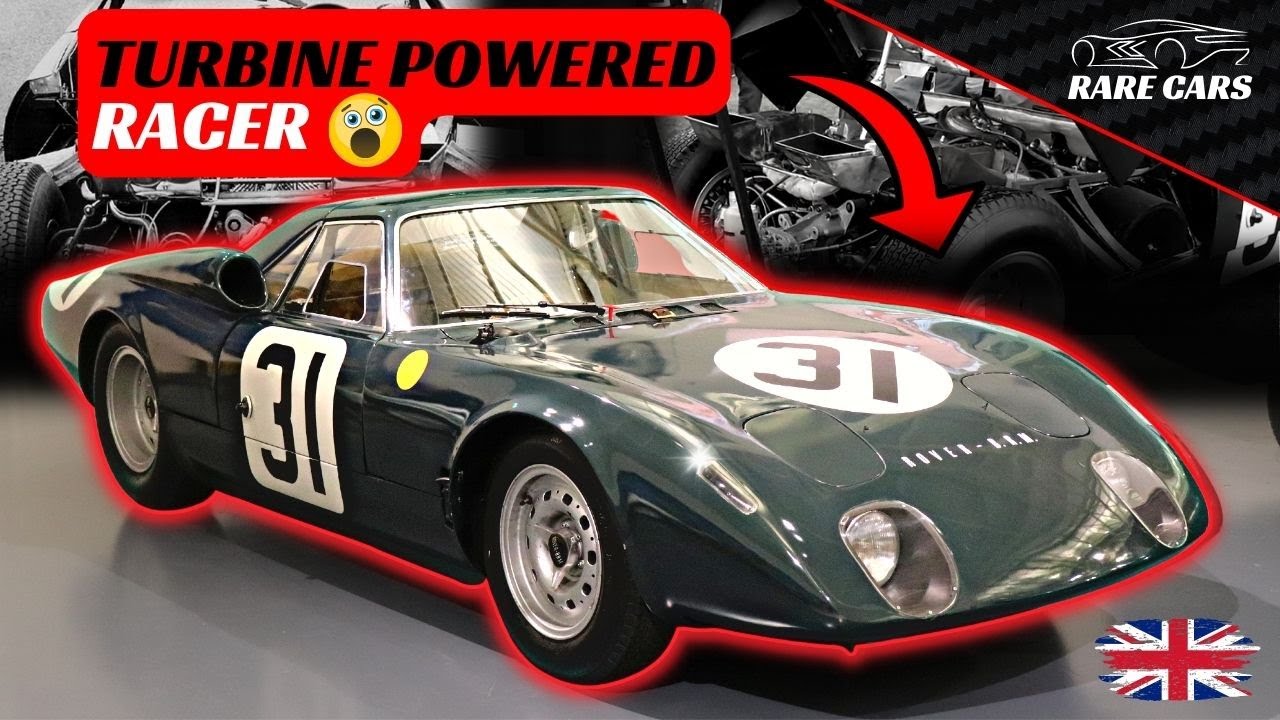The image features a sleek, dark green sports car designed for racing, prominently labeled with the number 31 on both the door and the hood, where it is placed diagonally within a circle. The car is outlined in red, adding to its striking appearance. The vehicle boasts thick black rubber wheels with steel hubcaps and four front lights, two of which are discreetly embedded into the car's surface. Above the car on the left side, a red text box with black lettering and a shocked-face emoji declares "Turbine Powered Racer." The top right corner of the image displays "Rare Cars" along with a white outline of a fast-moving vehicle. In the bottom right corner, a British flag is present, indicating the car's origin or relevance. Additionally, the image shows two smaller photos behind the main one, highlighting the car's internal mechanics and rear axle, suggesting it's part of an advertisement or informational display.